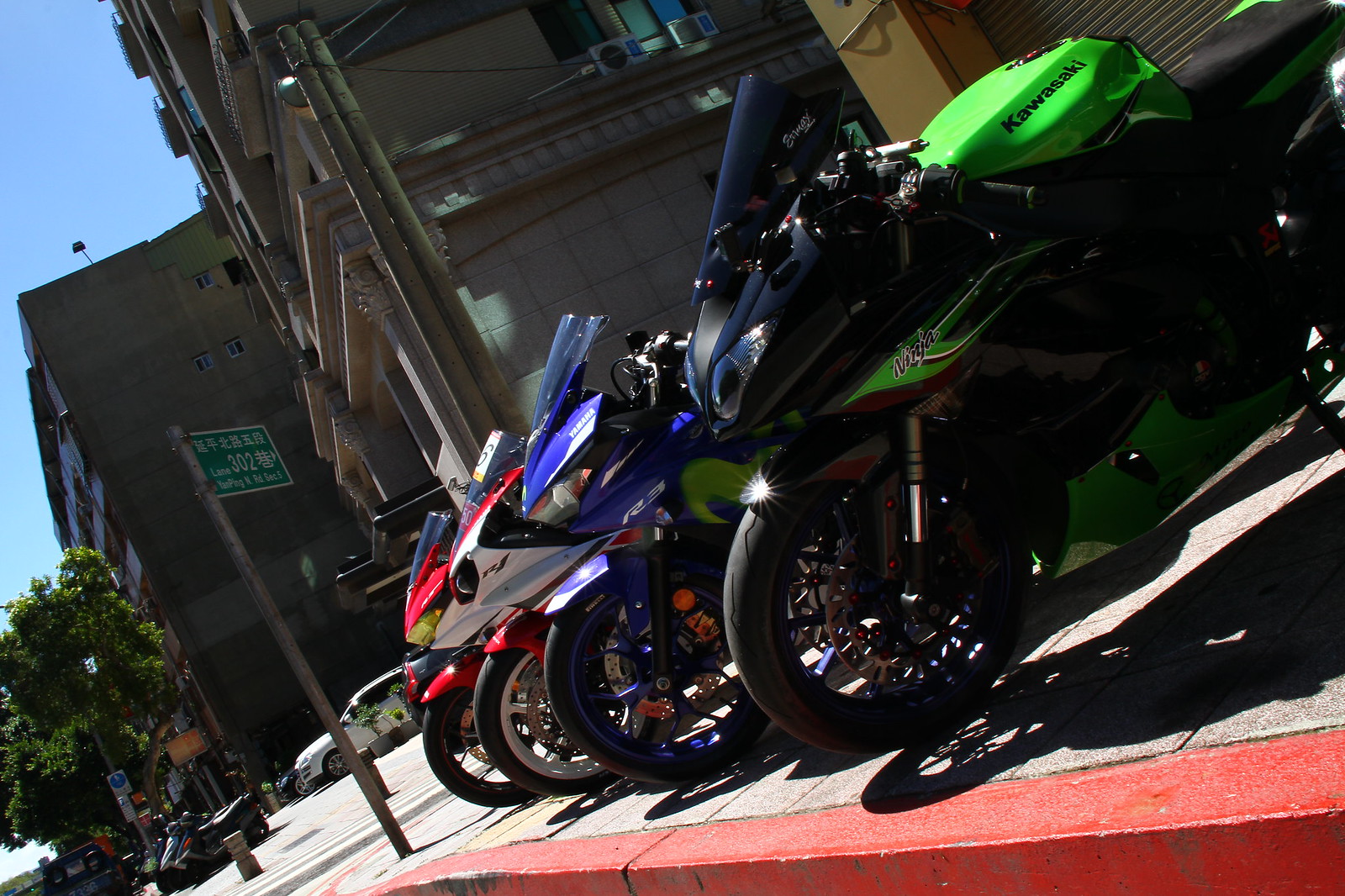This photograph captures a vibrant street scene featuring four sport motorcycles meticulously lined up at an angle on a gray cement sidewalk with a striking red curb. The first motorcycle in the foreground is a neon green Kawasaki Ninja, distinguished by its green fuel tank and black accessories, complemented by green pinstriping and a tinted windscreen. Following the Kawasaki, there's a blue Yamaha R3 with a black frame, succeeded by a white motorcycle with red accents, and finally, a red motorcycle with white accents at the rear of the lineup. The motorcycles, characterized by their angular styling and aggressive fairings, cast shadows on the pavement, indicating a sunny day under a clear blue sky.

The setting appears to be an Asian locale, suggested by a prominent street sign written in kanji, accompanied by the English text "Lane 302." This sign is mounted on a pole near the motorcycles. In the background, the scene is framed by multiple buildings, including a brown structure with cream-colored tiles and a larger gray and white stone building with three to four stories. A few trees and additional motorcycles or scooters can be seen across the street, along with a white car parked further down. The overall atmosphere portrays an urban environment bustling with life and activity.